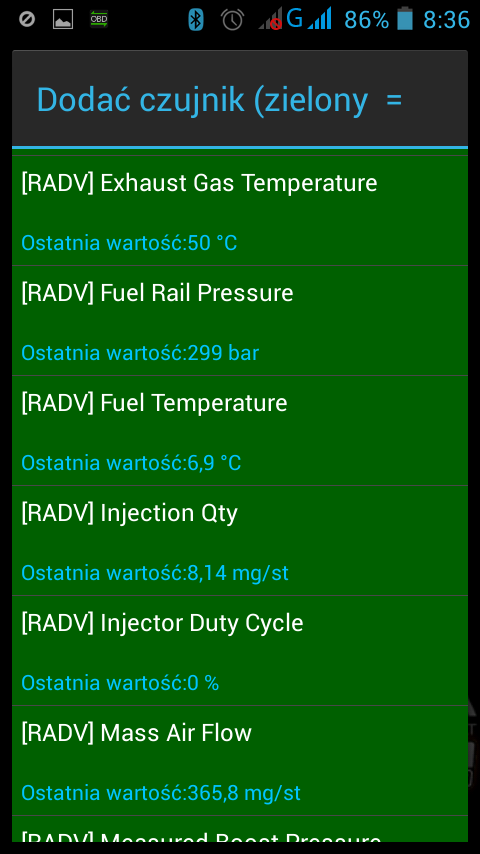This is a detailed screenshot of a mobile phone screen displaying a technical chart, likely related to automotive diagnostics. The top section features a notification bar with various icons indicating Bluetooth, alarm, signal strength, battery level at 86%, and the time, 8:36 AM. Below this, there's a grey horizontal strip with blue text in Polish, reading "Dodak CZUJNIK." The majority of the screenshot is characterized by a dark green background, containing a list of automotive parameters paired with their corresponding values. English text in white lists components such as "exhaust gas temperature," "fuel rail pressure," "fuel temperature," "injection quantity," "injector duty cycle," and "mass airflow." Each English term is followed by blue Polish text providing specific measurements: exhaust gas temperature at 50 degrees Celsius, fuel rail pressure at 299 bar, fuel temperature at 6.9 degrees Celsius, injection quantity at 8.14 mg/st, and so on. This comprehensive chart meticulously details essential engine components’ recommended temperatures, pressures, and quantities.